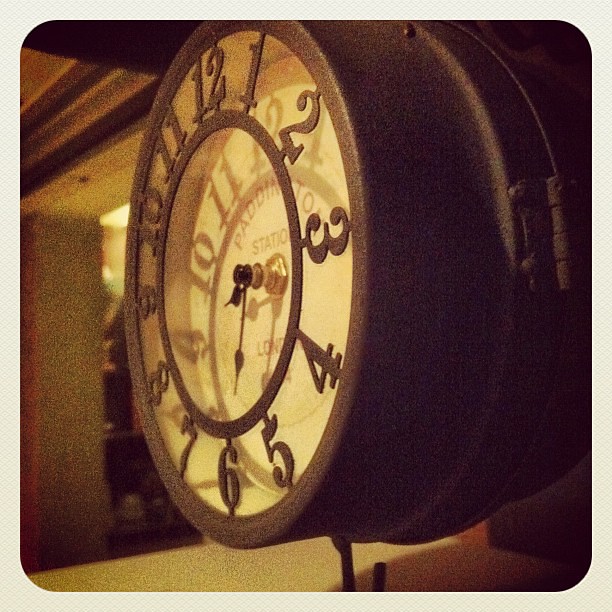The image features a vintage clock encased in a circular metal frame with a crosshatch-patterned border in a white-beige hue. The clock face, situated several inches deep within the frame, is white and prominently displays the inscription "Paddington Station, London." The numerals on the clock are affixed around the periphery and appear to be a bronzy color, while the clock hands are black and connected to a gold post. A hinge is visible on the bottom right side of the clock, possibly for opening and adjusting it. The time on the clock seems to be approximately 8:30.